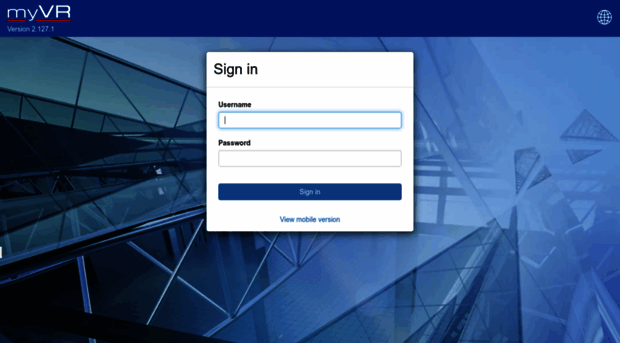This image is a detailed screenshot of a web page with an abstract design. At the top of the page, there is a prominent blue banner featuring the text "My VR" in white, which is underlined in red. Below this, although slightly blurry, it reads "version 2.127.1." On the right side of the same banner, there is a small white icon resembling a globe. 

The background of the web page displays a pattern consisting of varying shades of blue, seemingly depicting a structure with see-through walls and X-shaped designs on the sides. 

Superimposed on this background is a white sign-in box. The header of the box states "Sign In" in black text. Directly below are two input fields: the first is a blue bar labeled "Username" with a blinking cursor inside it, ready for user input, and the second is another bar labeled "Password" for entering the password. 

At the bottom of the sign-in box, a long blue button with the text "Sign In" in white awaits user interaction. Beneath this button, there is a link in blue text that reads "View Mobile Version."